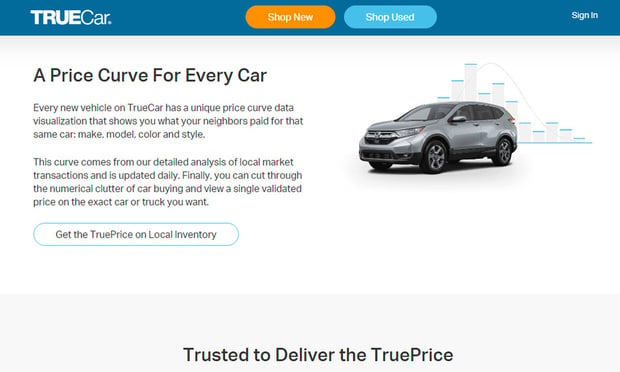This screenshot depicts a webpage with a clean, user-friendly interface. The background is predominantly white, highlighted by a slim blue header bar. In the upper left corner of this bar is the company's name, "TrueCar." Centrally positioned in the blue header is an inviting orange "Shop Now" button alongside a light blue "Shop Used" button. At the upper right corner, there is a clickable "Sign In" text for users.

Dominating the main section of the webpage is a striking image of a gray SUV, suggesting an example of the type of vehicles listed on the site. To the right of the SUV image, a simple graph illustration subtly emphasizes analytical data behind the pricing. Accompanying this visual, the text on the left outlines the service's unique selling proposition: "A price curve for every car." It elaborates that every new vehicle on TrueCar features a distinctive price curve data visualization, detailing the prices neighbors paid for similar cars in terms of make, model, color, and style. This pricing information is continuously updated from an in-depth analysis of local market transactions, aiding users in navigating car-buying decisions with a singular, validated price.

Below this informative content, a standout clickable button prompts users to "Get the True Price on Local Inventory," inviting them to explore specific listings.

At the bottom, a wide, extremely light gray footer spans the width of the page. Centralized within this footer, in bold black text, is the company’s tagline: "Trusted to Deliver the True Price." This footer encapsulates the value and reliability TrueCar promises its users.